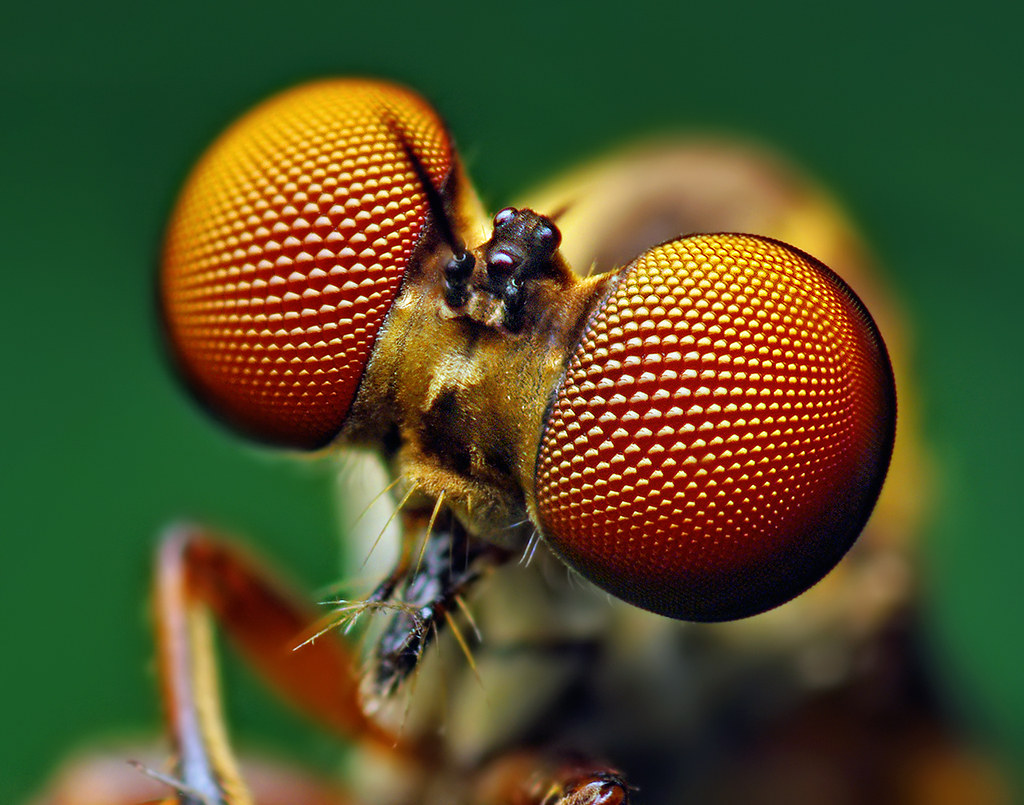This is an extremely close-up, crystal-clear photograph of an insect, showcasing its detailed facial features and intricate textures. Prominently displayed are two large, bulbous eyes positioned on either side of its head. These eyes are cylindrical in shape and exhibit a gradient of hues starting from a reddish-orange at the base, transitioning to a lighter orange, and finally to a burnt orange laced with black accents. The insect's head is adorned with golden and black accents, and features two antennae protruding outward. There is a noticeable black structure at the top of its head between the eyes, resembling a nose or mouthpiece. Fine golden hairs and additional black circles can be observed around the eye region. The insect's long, round legs are visible, with the left leg being more prominently displayed in the photograph. The background is green and blurred, ensuring all attention is drawn to the intricate and colorful details of the insect's head and body.